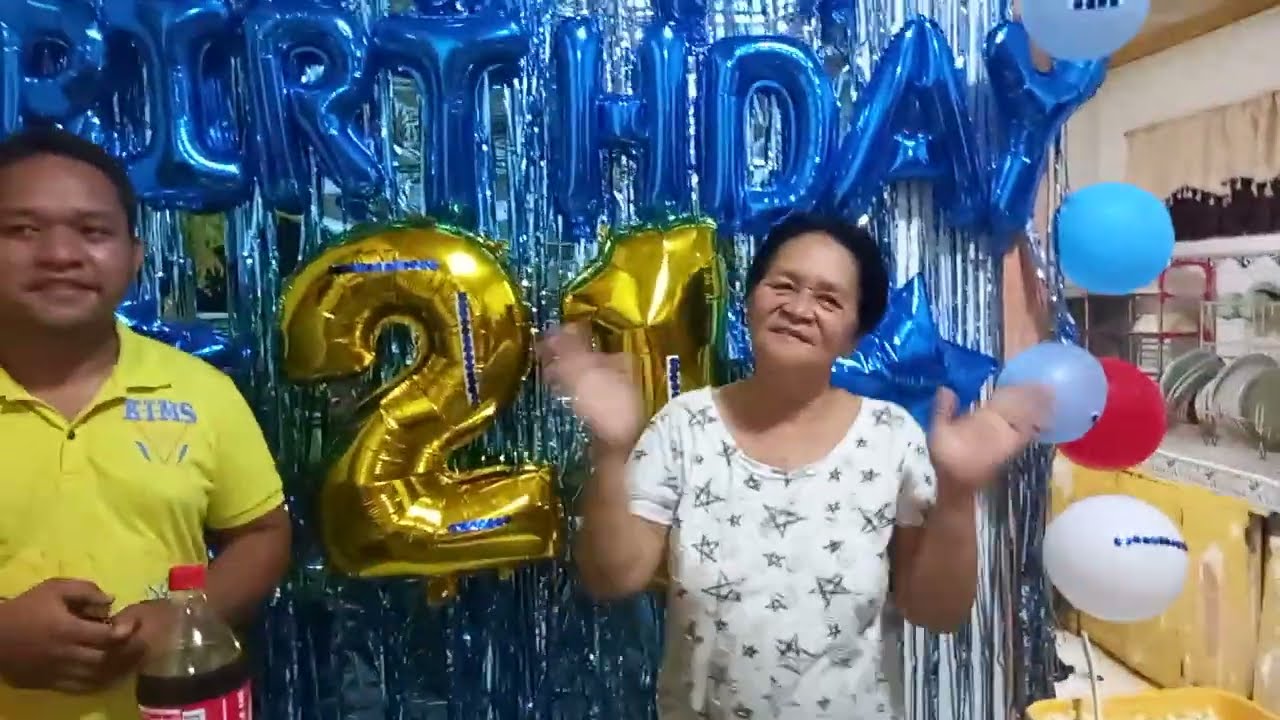The image captures a lively birthday celebration set in a room with blue tinsel garland streamers hanging vertically from the ceiling to the floor. The backdrop features mylar balloons spelling out "Birthday" in shiny blue letters, beneath which a gold balloon configuration displays the number "21." On the right side of this festive background, there are additional balloons in blue, red, and white, as well as a wall rack holding dishes and a small window.

In the foreground, two individuals stand prominently. To the left is a young man with brown skin and dark black hair, possibly of Pacific Islander, Hispanic, or Asian descent. He is dressed in a short-sleeved yellow polo shirt with the text "K-I-M-S" in blue, and has his hands cupped in front of his stomach. A partly visible two-liter Coca-Cola bottle is in front of him.

Slightly to the right of center is an older woman, who could be Filipino or Vietnamese. She has brown skin and dark hair, and she is wearing a white t-shirt adorned with black stars. With her hands raised and slightly blurred in motion, she appears to be clapping or making "jazz hands." The celebratory atmosphere, highlighted by the decorations and the interactions of the individuals, suggests that it is a special 21st birthday event.